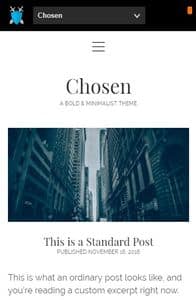The image features a predominantly white background with a black header at the top. The header contains white text and includes a search box with the word "chosen" inside it. On the top-left corner of the header, there is an icon of a blue shield crossed by two swords. 

The main section of the page has a white background with text written in black and blue. The word "chosen" appears prominently in blue but is slightly blurry. Central to the page is a dark blue-toned image of buildings occupying the middle, left, and right sides.

Below the image, the text "This is a standard post" appears clearly in black, followed by a statement at the bottom of the page, "This is what an ordinary post looks like. And you are reading a custom, except right now," also in black text. Despite some blurriness in the text, it remains legible. Key phrases like "chosen," "this is a standard post," "this is what an ordinary post looks like," and "you are reading a custom, except right now" are written in larger font sizes.